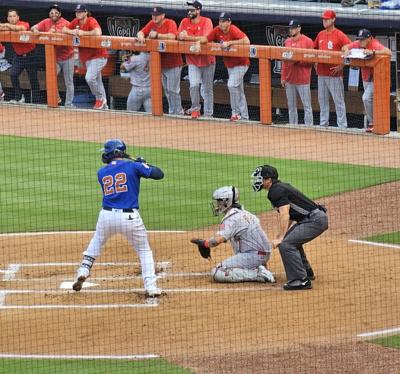The image captures a detailed moment of a baseball game, potentially a Major League Baseball event, taken from a perspective slightly behind the netting, close to the third baseline. In the foreground, we have a batter clad in a blue jersey with the number 22 in red on his back and white pants, preparing to swing with his bat resting on his shoulder and his front foot slightly lifted. Positioned behind him, the catcher is in a gray uniform, equipped with a baseball mask and protective pads on his knees and chest. The umpire, wearing black shirt and gray pants, crouches behind the catcher, poised to make a call. The home plate is clearly visible, surrounded by a large dirt circle with distinct white chalk lines. In the background, within the dugout, all players are dressed in red or orange tops, implying them as the opposing team. The dugout is marked by an orange guardrail, adding a splash of color to the scene ornamented by well-maintained grass. The high-quality equipment and the meticulous field grooming further underscore this as a professional game setting.